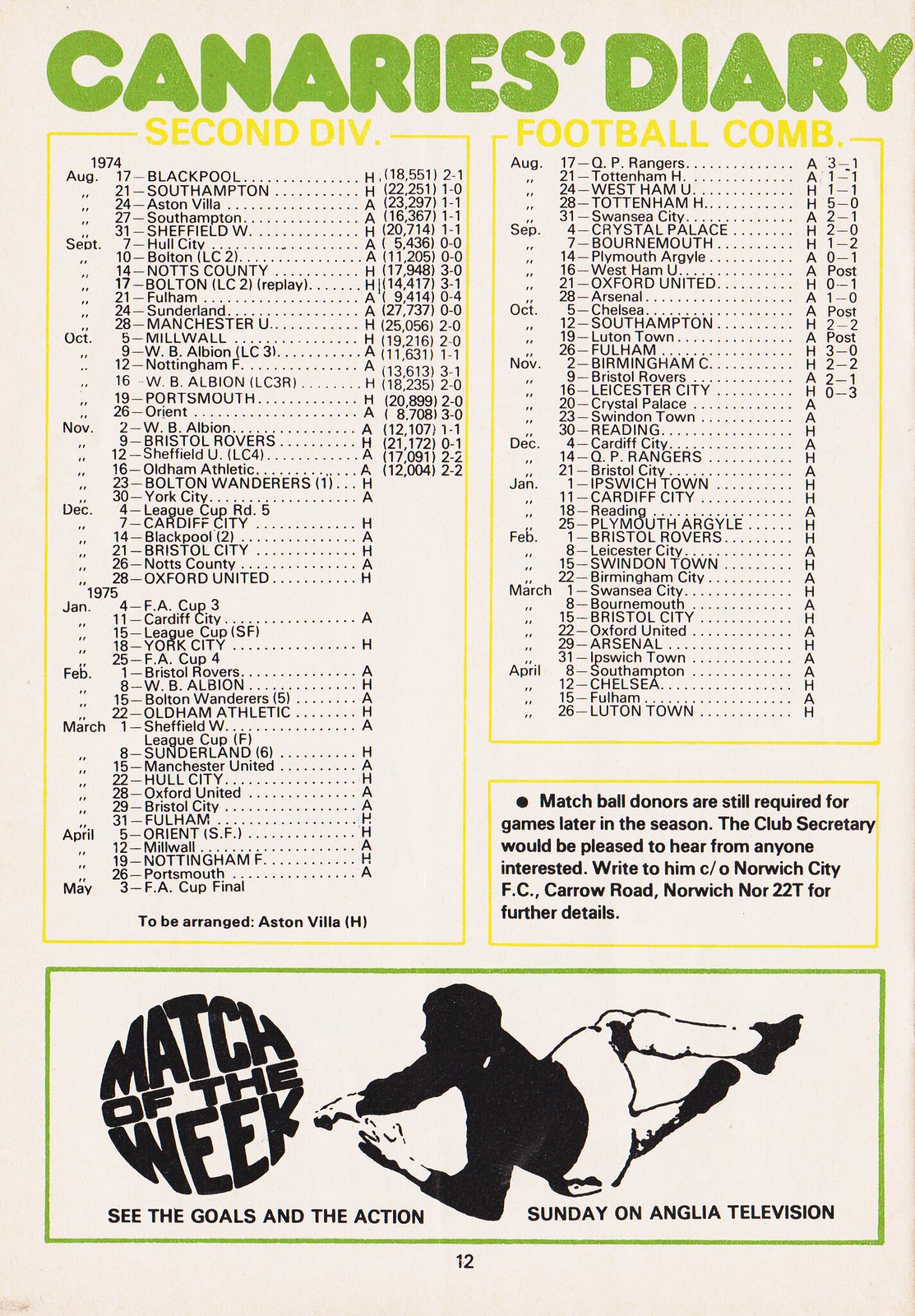The image depicts a digital poster detailing the schedule for a sports team event. At the very top, it features the title "Canaries' Diary" prominently in big green letters. Below this title, the content is divided into two main columns. The left column is titled "Second Div." bordered in yellow, and contains a schedule with dates, team names, and numbers listed in black text. The right column, titled "Football Comb." also in yellow, lists similar structured details with dates, names, letters, and numbers. Underneath the "Football Comb." column, there is a small yellow rectangle with around six lines of black text involving administrative or additional notes.

Towards the bottom of the poster, there's a green-outlined rectangle. Inside this rectangle, on the left side, the words "Match of the Week" are stylized in a circular shape resembling a bowl. Adjacent to this text is a black and white drawing of a soccer player diving to the left. Below, it reads "See the Goals and the Action Sunday on Anglia Television." The background of the entire poster is white, and the primary colors used are green, yellow, and black. At the very bottom center of the page, there is a small black number "12.” Overall, it visually conveys the event schedule and additional announcements related to a soccer team in a structured and colorful manner.